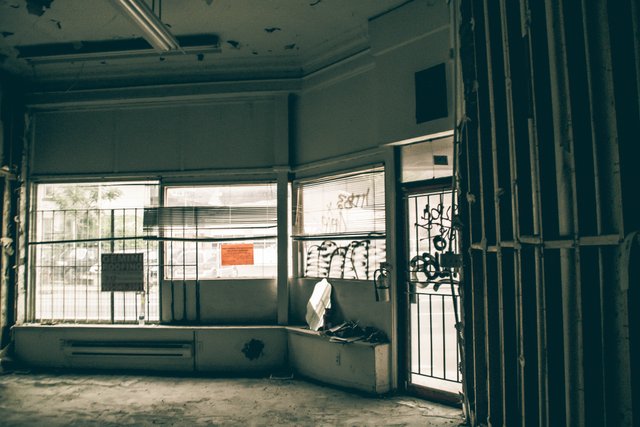The image depicts an indoor scene of an abandoned store with a vintage filter effect. Dominated by a dull green hue, the setting features a wall with windows and a door, both secured with bars and marked by graffiti. The windows have partially drawn blinds and display an orange sign, along with another sign that reads "Gemini Roofing," though the other text remains unreadable. Inside, the floor is dirty and torn up, resembling worn tile or cement, and a baseboard heater is attached below the windows. The ceiling shows signs of peeling paint, adding to the overall dilapidated atmosphere. Debris scattered on the windowsill and the absence of furnishings or any significant color reinforces the neglected state of the space. The light entering the room solely comes through the barred windows, casting a muted glow over the scene.